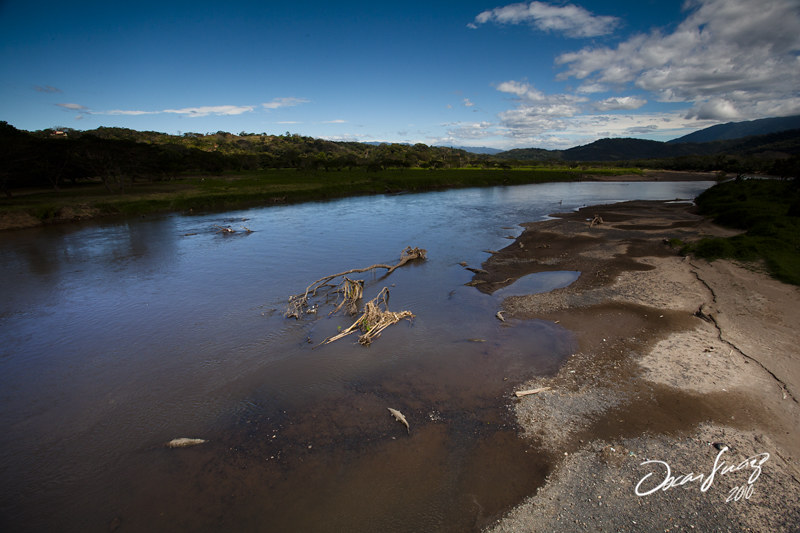This detailed and vibrant image captures a river flowing from the lower left corner and winding towards the upper right. On the right side, there is dry land interspersed with sand, stone, and a coronary plant. Notably, the river transitions from blue to brown and murky as it nears the shore, covering the rocks. Additionally, there are fallen trees extending into the water, and a brown tree branch lying in the river's center. The bottom of the image features what appear to be two fish; one on the bottom left and another in the bottom center.

A signature reading "Oscar Suaz 2010" is inscribed in the lower right corner, marking the photograph's creation date. The upper part of the image reveals a serene landscape with low, shadowy mountains and a granary field adorned with trees. A solitary house is visible on the upper left. Beyond the mountains, a blue sky with scattered white clouds further enriches the scene. A noticeable crack runs through the ground on the image's right side, adding an element of ruggedness to the picturesque view.